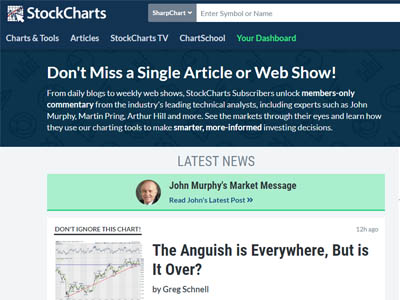The image is a meticulously organized informational block, presented in a square format. The top half of the square showcases a dark blue background, while the bottom half features a predominantly white background with a thin horizontal strip of light blue-green.

At the upper-left corner of the dark blue section, the text "Stock Charts" is prominently displayed. Adjacent to this title, a search prompt states, "Sharp chart, enter symbol or name." Below this, a horizontal navigation menu lists several categories: "Charts and Tools," "Articles," "Stock Charts TV," "Chart School," and "Your Dashboard." The first four labels appear in white, whereas "Your Dashboard" is highlighted in green, indicating the current selection.

Beneath the navigation menu, a promotional section in white text states, "Don't miss a single article or web show. From daily blogs to weekly web shows, Stock Charts subscribers unlock members-only commentary from the industry's leading technical analysts, including experts such as John Murphy, Martin Pring, Arthur Hill, and more. See the markets through their eyes and learn how they use our charting tools to make smarter, more informed investing decisions."

Directly below, a heading labeled "Latest News" introduces two featured content blocks. The first block includes an avatar of an older Caucasian gentleman with a bald head smiling, alongside the caption, "John Murphy's Market Message. Read John's latest post."

Adjacent to this, on the left side, a small bar chart graph is labeled "Don't ignore this chart." To the right of this graph, another news snippet reads, "The anguish is everywhere, but is it over?" by Greg Schnell, posted 12 hours ago.

Overall, the image clearly delineates the structure of information, prioritizing readability and user-friendly navigation.